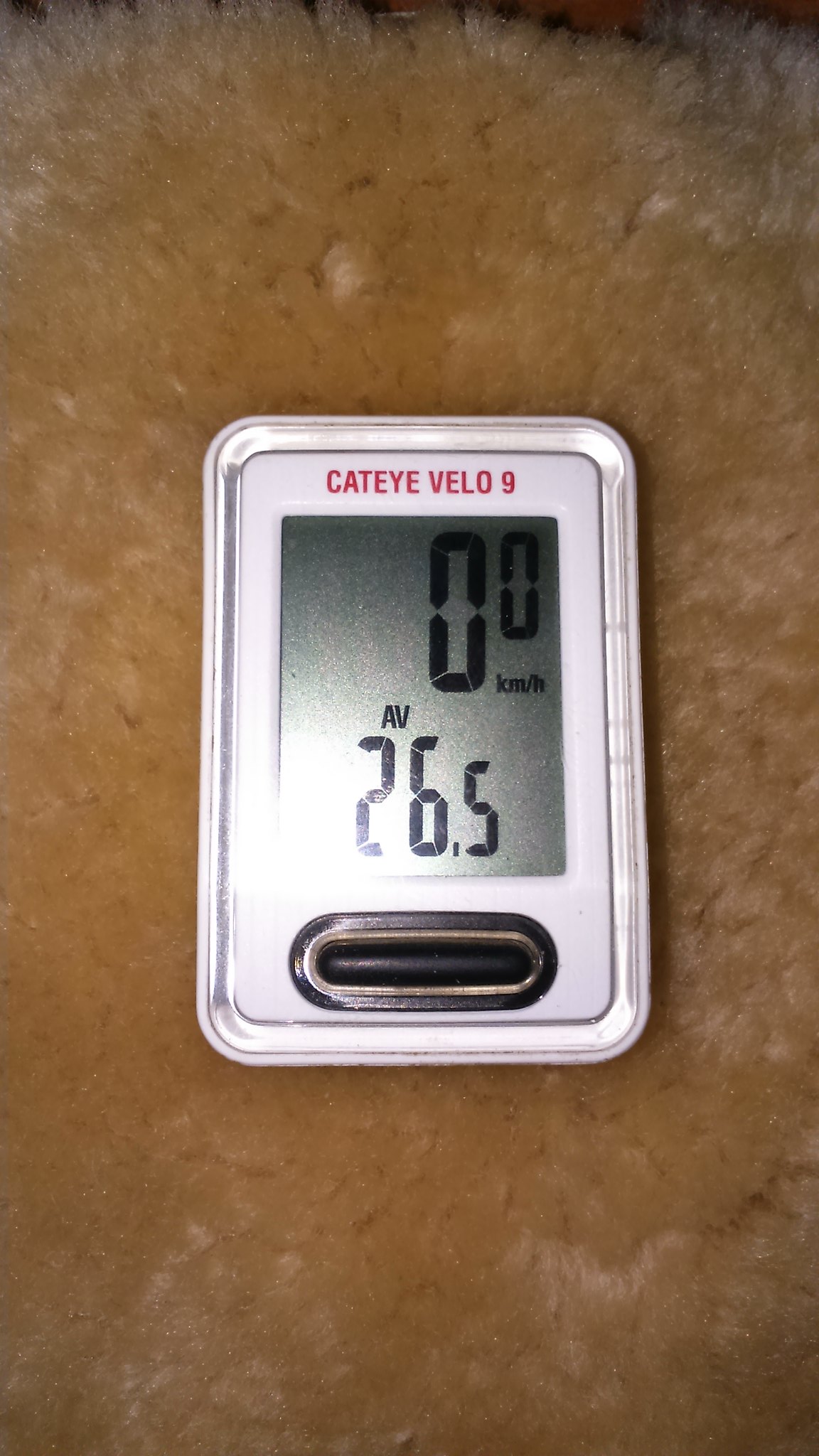This photograph depicts a small, rectangular device resembling a step tracker. The device is predominantly white with a silver outer shell. At the top, "Cat Eye Velo 9" is prominently displayed in red text. The device features an LED screen, where the top section shows the number "0" with a "0" in the exponent position. On the bottom right of this number, "km/h" (kilometers per hour) is indicated, suggesting it measures speed. Below this, "AV 26.5" is displayed, though its exact meaning is unclear; it could possibly refer to an average speed or another metric. At the bottom of the device, there is a black, oval-shaped slot, which seems designed for an insertable component. The device is placed on a surface that is brown and white, hinting that the photograph might have been posted on social media, perhaps showcasing the results of an experiment or a recent journey.